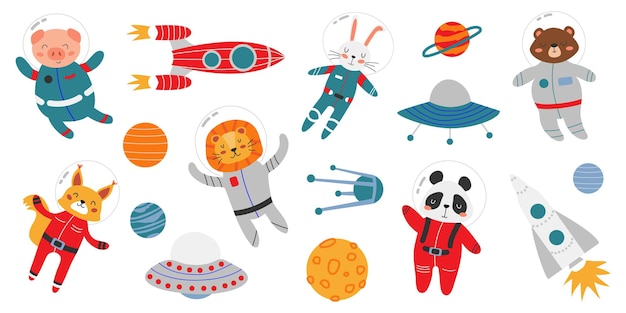This charming illustration features a group of adorable animal characters dressed as astronauts, each donning vibrant spacesuits. A little pig and a white bunny shine in turquoise suits, matching perfectly. A bear and a lion coordinate in gray, while a spunky fox and an endearing panda sport red spacesuits. All characters wear astronaut helmets, adding to the space adventure theme. The scene is enriched with a red rocket, a white rocket, and two UFOs. Around them are various planets of different sizes, including a recognizable Saturn with its iconic ring. Dominating the center of this whimsical space utopia is a little satellite, anchoring the entire delightful composition. This cute and cohesive image uses a well-harmonized color palette and showcases humanoid-like animals, emphasizing their shared adventure in a fantastical space setting.